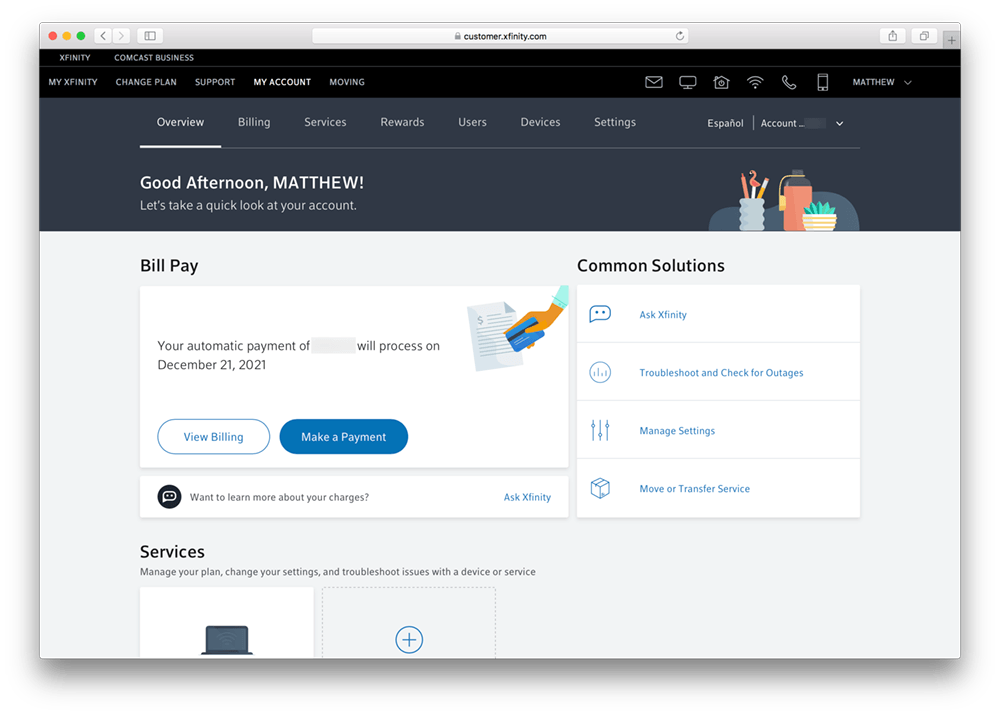**Detailed Caption:**

The image appears to be a mock-up of someone using a Mac web browser, evident from the presence of a large drop shadow, which suggests it is not an actual screenshot but possibly a screenshot of a screenshot. At the top, the browser chrome displays the URL "customer.xfinity.com".

The webpage features a black header with the logos "Xfinity" and "Comcast Business". On the left side of the black menu, there are several options listed: "My Xfinity", "Change Plan", "Support", and "My Account" (which is highlighted in white), followed by "Moving". Icons on the right include an envelope, a screen, a house, a beacon, a phone, and a smartphone. A dropdown menu with the text "Matthew" is also visible.

Beneath the main menu, a gray submenu lists different sections: "Overview" (highlighted), "Billing", "Services", "Rewards", "Users", "Devices", "Settings", and "Español". The account section appears grayed out.

Below the gray menu, the text "GOOD AFTERNOON, MATTHEW" is displayed in all caps, accompanied by the phrase "Let's take a quick look at your account". The right side of the screen shows a simple graphic of pencils, a water bottle, and a plant on a desk.

The main content area is divided into sections. On the left, under the header "Bill Pay", there's a notification about an automatic payment scheduled for December 21, 2001, with the original payment date crossed out. Below are buttons labeled "View Billing" (white) and "Make a Payment" (blue).

On the right, under "Common Solutions", options include "Ask Xfinity", "Troubleshoot and Check for Outages", "Manage Settings", and "We Transferred Service", each accompanied by icons.

Further down, another section labeled "Services" allows users to manage their plans, change settings, and troubleshoot issues. This includes a laptop graphic with a plus arrow suggesting additional details or actions can be accessed.

Overall, the mock-up offers an extensive, user-friendly overview of account management features and customer support options available on Xfinity’s website.